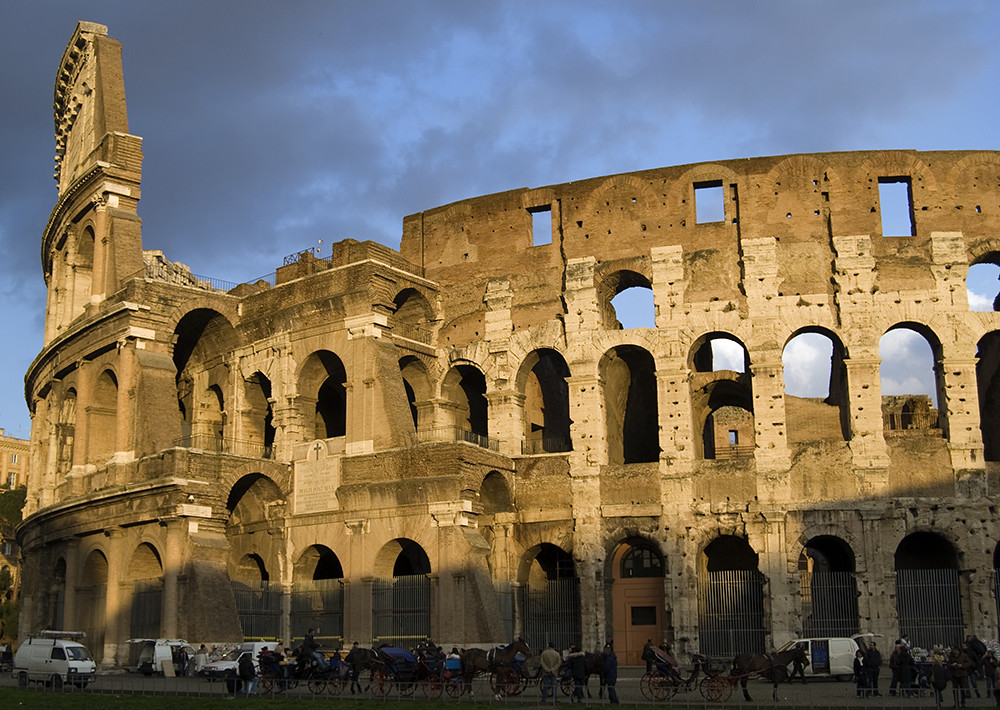This photograph captures a vibrant outdoor scene featuring the historic Roman Colosseum. The sky is a mix of blue and dark gray clouds, casting dynamic shadows and illuminating the ancient structure. The Colosseum, a circular stone amphitheater with three rows of arched doorways, is prominently displayed with sunlight highlighting its upper sections. Despite its age, the Colosseum is remarkably well-preserved, with only the top areas showing some darker discoloration.

The busy scene at the bottom is filled with tourists and bustling activity. Numerous people can be seen capturing photos, exploring, and lining the streets near street markets and vendors. The area is populated with various vehicles, including several white vans, trucks, and cars, alongside a dozen horses. The ambiance of historical splendor and contemporary life melding together is encapsulated by the steel, spear-shaped fences, large wooden doors, and the vibrant presence of visitors experiencing the rich history of the Colosseum. Through the open arches of the Colosseum, the blue sky and drifting clouds add a timeless backdrop to this captivating image.